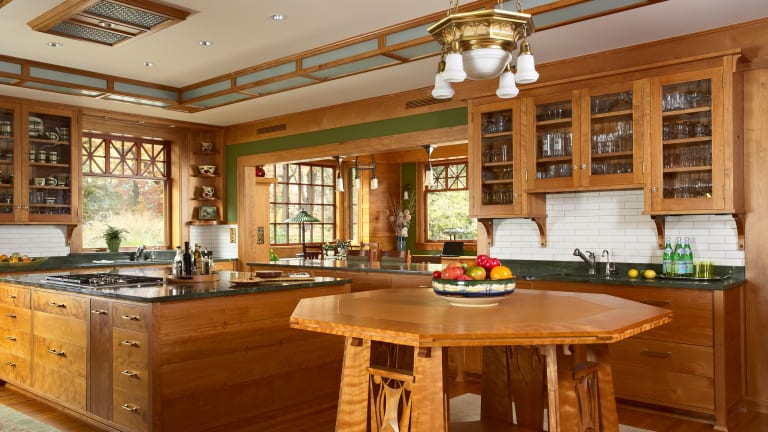The image depicts a spacious, modern-country kitchen characterized by abundant light pine wood surfaces, contrasting black countertops, and a harmonious blend of functional and decorative elements. The white ceiling features perimeter lighting and a central vent, bordered by brown trim with blue glass accents running along the right side and the back. A chandelier with gold and milk glass lights hangs prominently, providing a focal point of elegance. 

Dominating the center of the kitchen is a large wooden island with a polished black marble top. This island boasts multiple drawers with bronze handles, a streamlined sink, and a tray holding an assortment of spice bottles. Against the back wall, a series of cabinets with glass fronts reveal neatly arranged dishes and glasses. Below these cabinets, the area with a tile backsplash showcases a silver faucet and a gleaming sink, accompanied by three green glass bottles and two lemons.

To the right, in the corner, three small shelves host an array of decorative teacups. A large window trimmed in pine allows natural light to flood in. Adjacent to this, a wide opening leads to another room, visibly holding a table and more windows. The border of this opening is green with a top layer of brown wood, blending seamlessly into the kitchen's overall aesthetic.

A notable hexagon-shaped table with wide pine legs stands in front of the island, partially topped with black. A black-and-white pottery bowl filled with colorful fruits—red, orange, and green—sits at its center. The kitchen exudes warmth and functionality with a harmonious blend of wood, glass, and natural elements, accentuated by thoughtful lighting and decor.